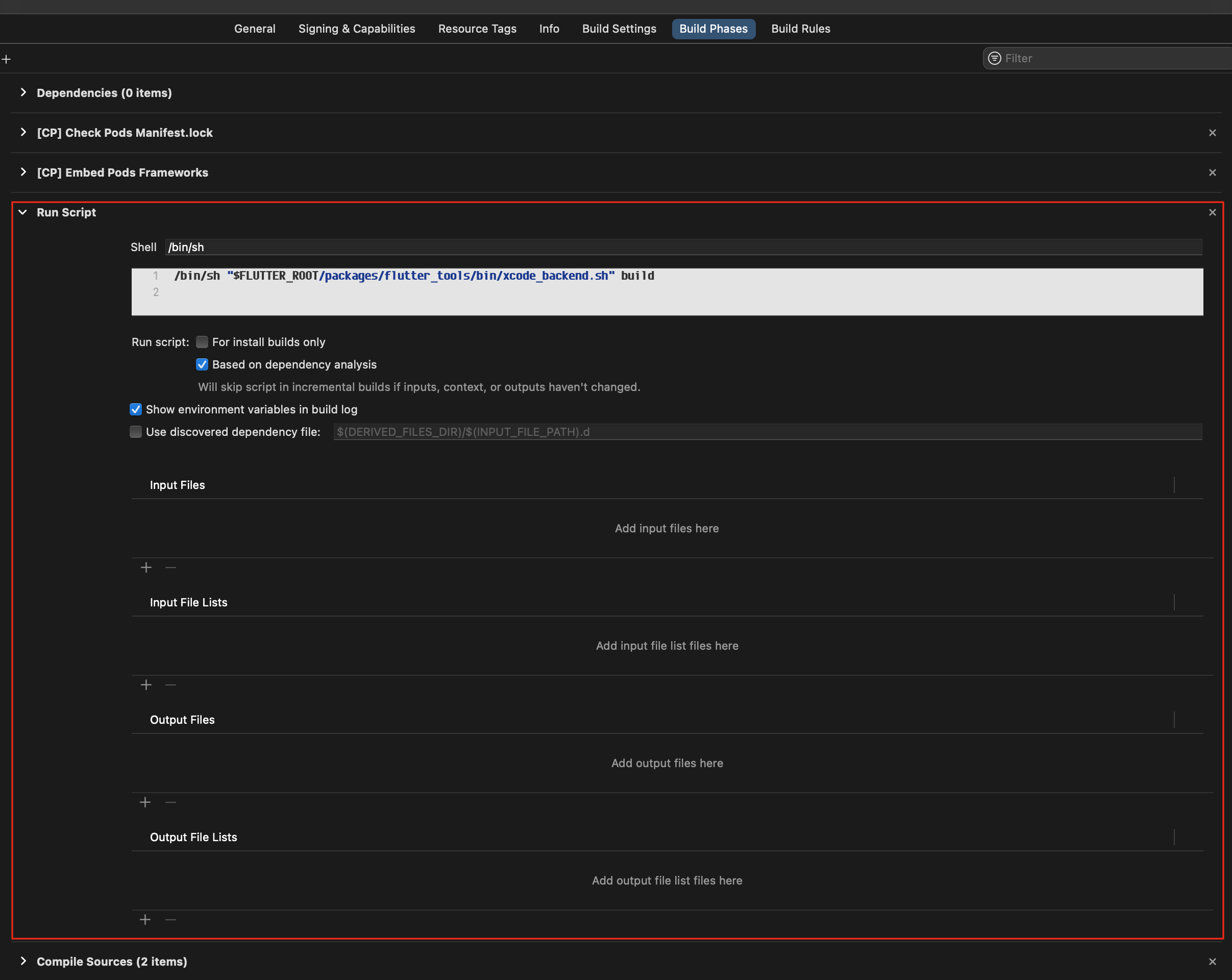The image depicts a detailed interface of a software development environment, presumably for coding or compiling software. The entire scene is set on a dark gray or black background, giving it a sleek and modern appearance. The top section features a long, thin black rectangle that contains seven buttons, each labeled with white text, indicating different settings categories. The highlighted button, "Build Phases," is surrounded by a blue rectangle, making it stand out. The categories, in order from left to right, are: General, Signing & Capabilities, Resource Tags, Info, Build Settings, Build Phases, and Build Rules.

Beneath this, there is another narrow black bar on the far right side containing a dark gray text box labeled "Filter." This row also features three drop-down buttons: Dependencies, Check Pods Manifest, and Embed Pods Frameworks. Below this, the "Run Script" drop-down menu is open, revealing multiple options.

The first row in the "Run Script" section shows a line of code within a long, white rectangular input field. Directly below this input field, there is another "Run Script" label, followed by various buttons for executing the script. Additionally, there are multiple fields for inputting files, providing a comprehensive view of the customization and build configuration options available within the software.